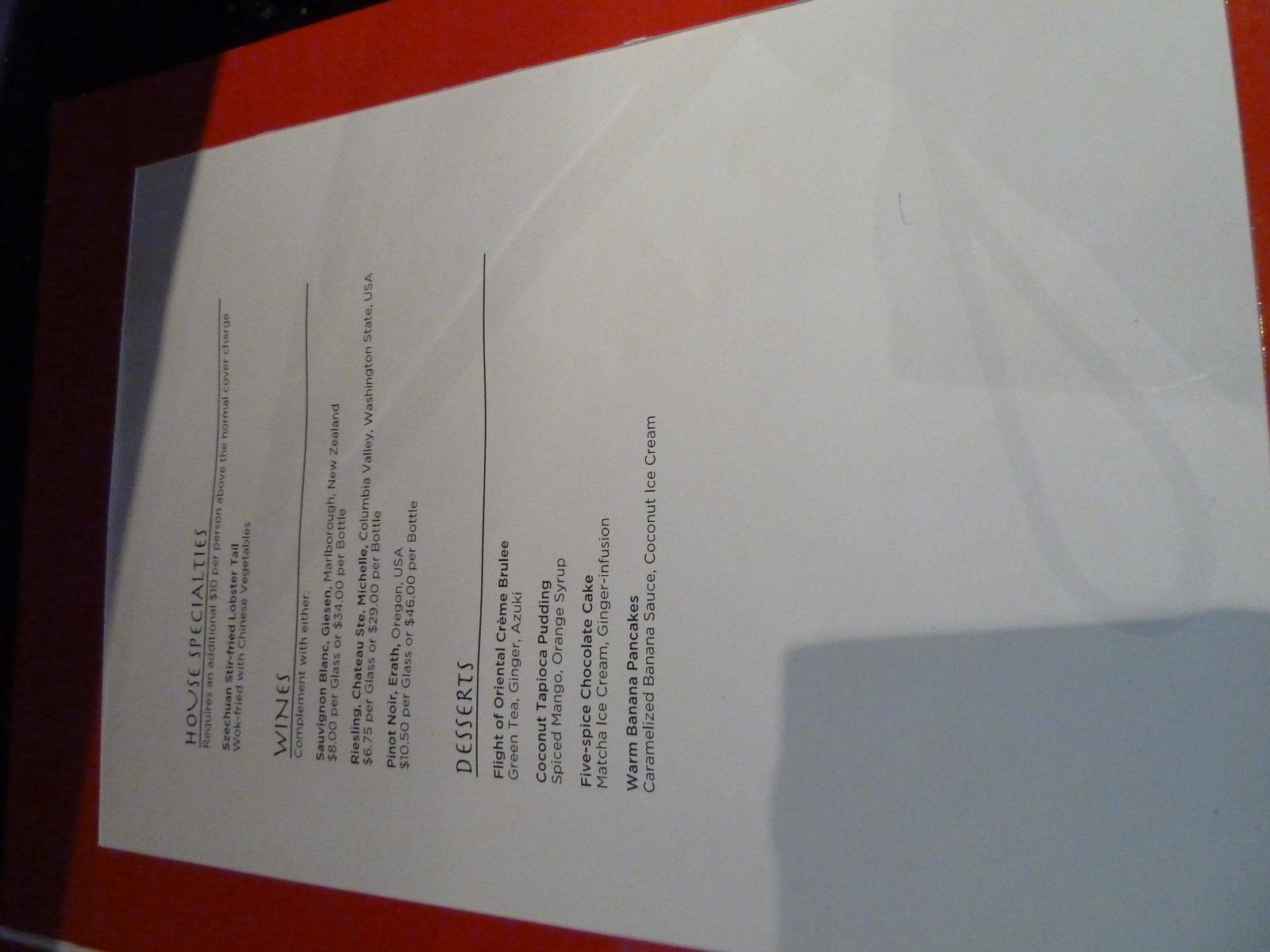The image displays a vertically oriented section of a menu printed on white paper with black text, the content aligned to the left side. At the top, the heading reads "House Specialties," which requires an additional $30 per person above the normal covered charge. Listed under this section is the dish "Szechuan Stir-fried Lobster Tail," described as wok-fried with Chinese vegetables.

Following this, there is a section titled "Wines," suggesting pairings to complement the meal. The options include:
- Sauvignon Blanc from Gießen Marlborough, New Zealand, priced at $8 per glass or $34 per bottle.
- Riesling from Chateau St. Michelle, Columbia Valley, Washington State, USA, priced at $6.75 per glass or $29 per bottle.
- Pinot Noir from A to Z, Oregon, USA, priced at $10.50 per glass or $46 per bottle.

The menu then lists "Desserts" with the following options:
- Flight of Oriental Crème Brûlée featuring Green Tea, Ginger Azuki, Coconut Tapioca Pudding paired with Spiced Mango Orange Syrup.
- Five Spice Chocolate Cake.
- Matcha Ice Cream with a Ginger Infusion.
- Warm Banana Pancakes served with caramelized banana sauce and coconut ice cream.

The text extends about halfway down the page, providing a detailed view of the restaurant's specialty offerings, wine suggestions, and dessert choices.